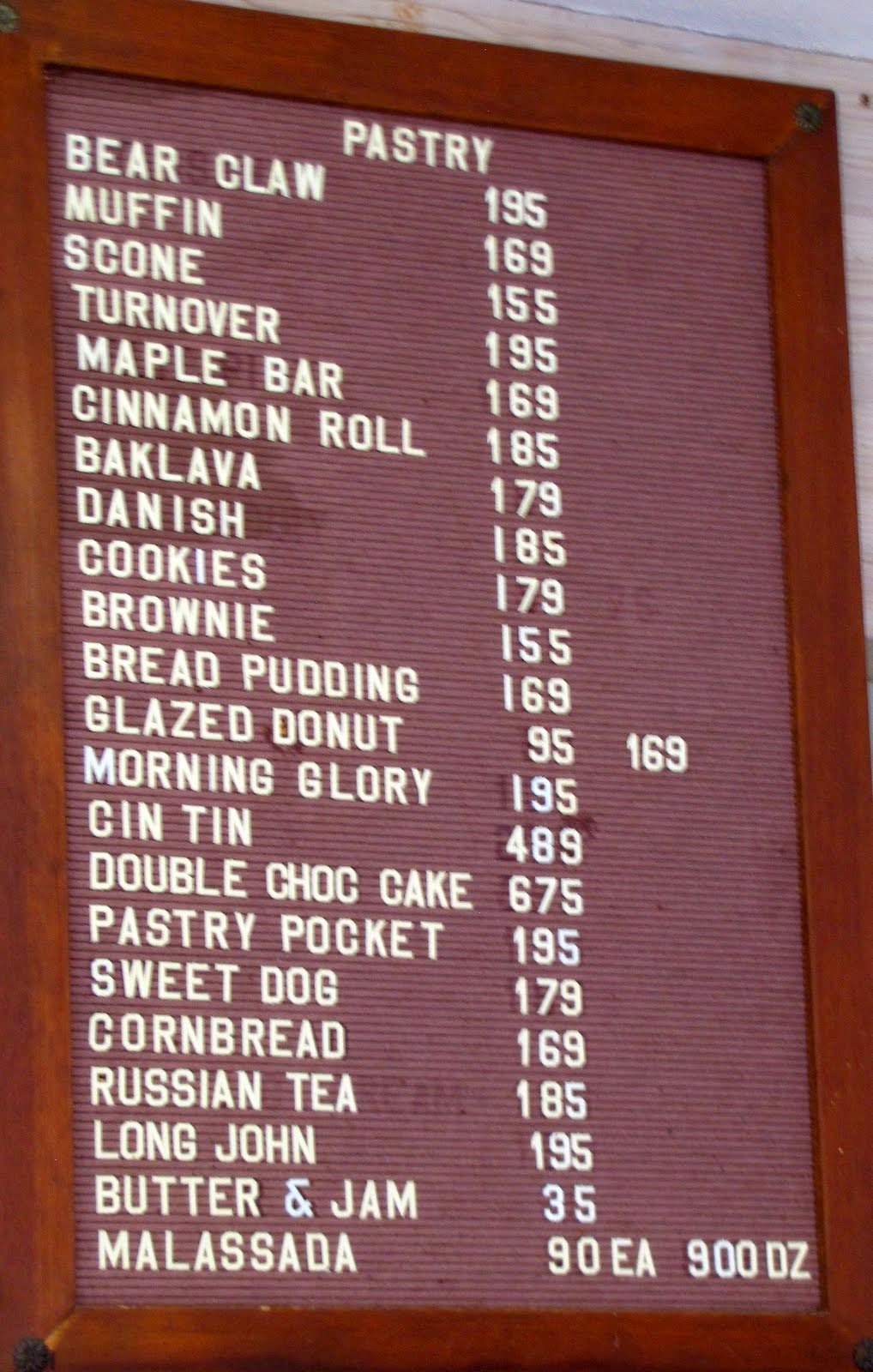This photograph showcases a large, vertically-oriented felt board menu, meticulously nailed to a wooden wall, with a sliver of the wall barely visible at the top right corner. The board's wooden frame contrasts elegantly with its soft pink felt background, providing a charming, rustic touch. The menu is adorned with crisp white text listing an array of pastries and their prices, neatly organized to tempt any passerby. 

Offerings feature:
- Bear Claw: $1.95
- Muffin: $1.69
- Scone: $1.55
- Turnover: $1.95
- Maple Bar: $1.69
- Cinnamon Roll: $1.85
- Baklava: $1.79
- Danish: $1.85
- Cookies: $1.79
- Brownie: $1.55
- Bread Pudding: $1.69
- Glazed Donut: $1.95, $1.69
- Morning Glory: $1.95
- Sin Tin: $4.89
- Double Chocolate Cake: $6.75
- Pastry Pocket: $1.95
- Sweet Dog: $1.79
- Cornbread: $1.69
- Russian Tea: $1.85
- Long John: $1.95
- Butter and Jam: $1.35
- Malasada: $0.90 each, $9.00 per dozen

The meticulous arrangement and diverse selection make this menu board both visually appealing and appetite-inducing, capturing the warmth and charm of a cozy bakery.